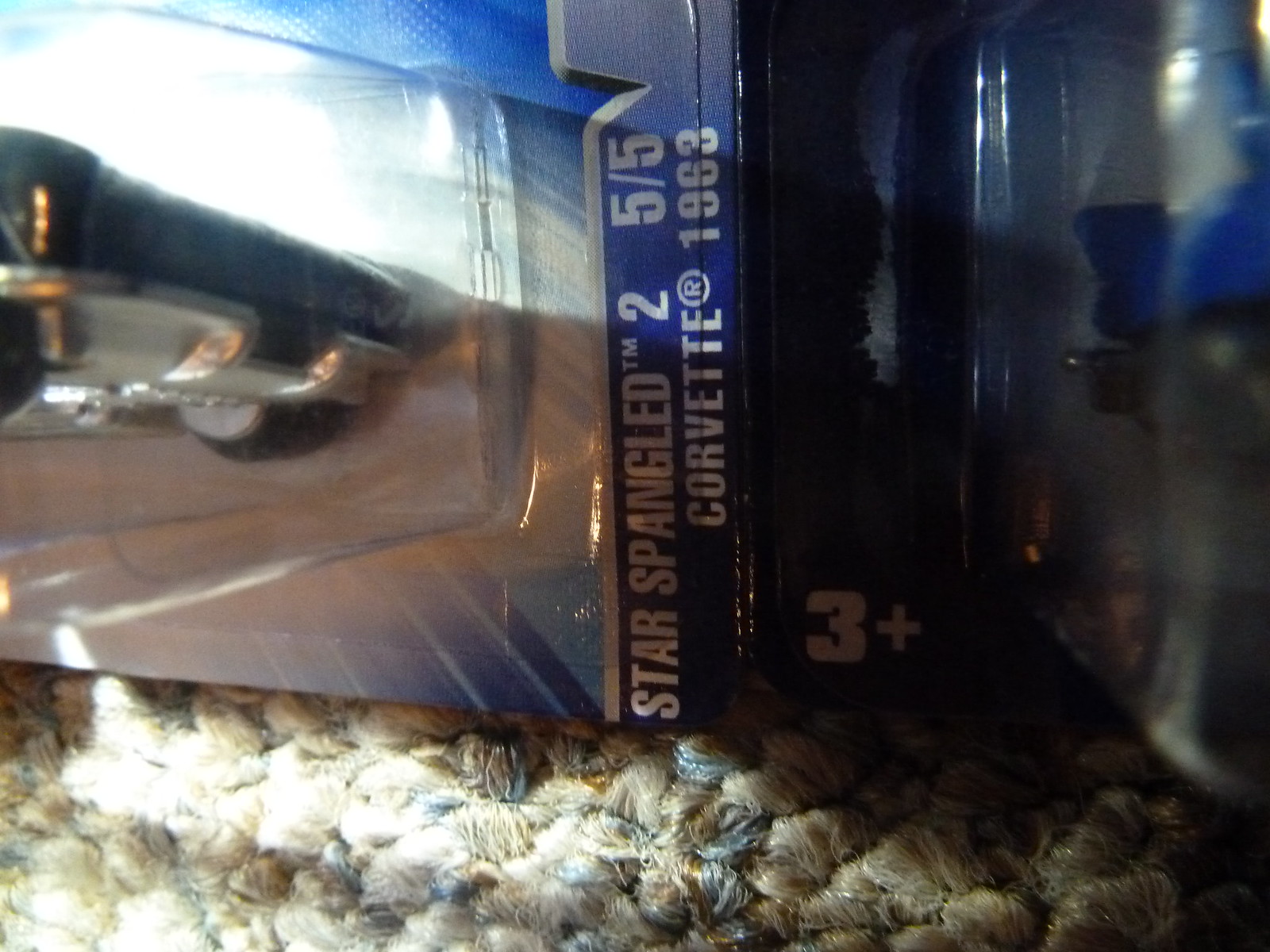The image features a close-up view of a rectangular object, likely a packaged product, placed on a woven mat. The scene is illuminated by a light source, creating a play of shadows and highlights across the item. The primary colors visible are shades of tan, beige, and gray, contributing to a textured and nuanced appearance. The product is encased in a blue and clear plastic package, adorned with white lettering that runs sideways. Prominently displayed on the packaging are the details: “For ages 3+,” "Star Spangled 2," and a rating of "5 out of 5." Additionally, the package specifies the item as a "Corvette 1963." The packaging appears to have a peel-off plastic cover, hinting that it needs to be removed to access the Corvette model inside.